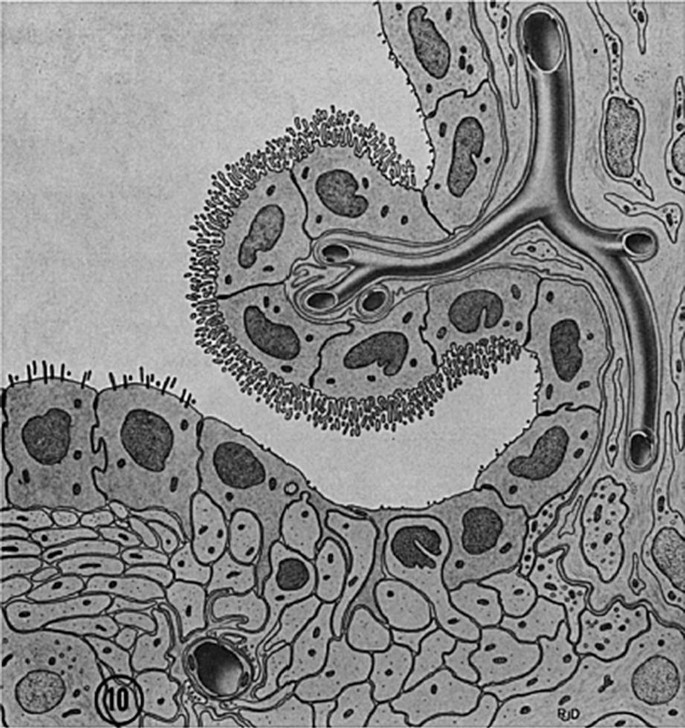This highly detailed black and white illustration appears to showcase a microscopic view of biological structures, likely showcasing a close-up of cellular and vascular features that could potentially belong to either a living organism or a plant. The image is meticulously drawn with various shades of gray highlighting multiple individual cells grouped together. Prominently in the middle of the image, extending towards the top right, are several tubular structures that resemble veins or other similar pathways. These tubes branch out, seemingly connecting to different clusters of cells. Notably, the illustration includes some small pores or hair-like extensions projecting from the cells or linings, which could be representative of cilia or similar structures. In the bottom left corner, a black circled number '10' is clearly outlined, standing out against the background, providing a unique identifier within the image.